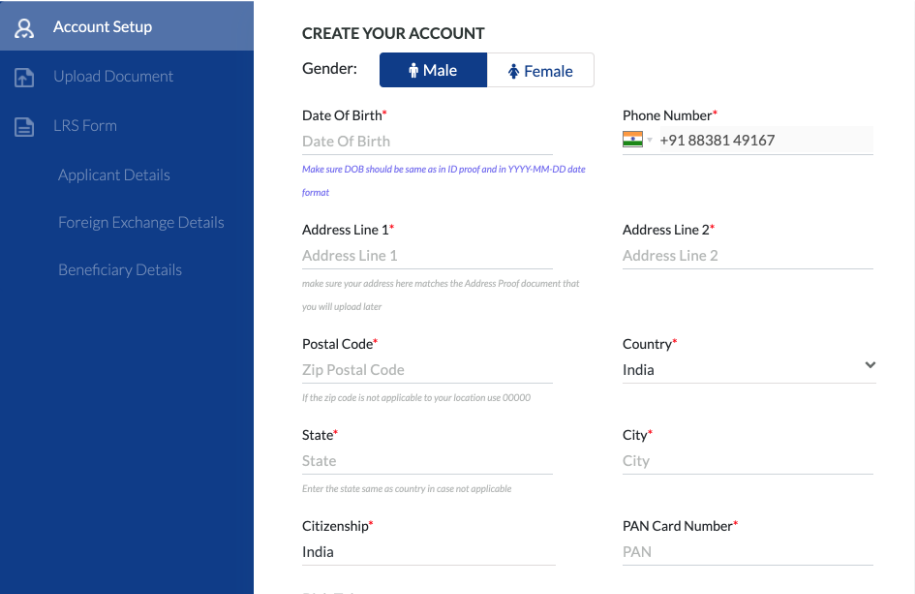A detailed descriptive caption for the image could be:

---

The image is a screenshot of a web page dedicated to account creation. On the left side, a vertically-aligned sidebar features a pleasant shade of royal blue transitioning to a lighter blue at the top. The header "Account Setup" is displayed prominently in a white font. Beneath this header, several options are listed in a light blue font: "Upload Documents," "LRS Forms," "Applicant Details," "Foreign Exchange Details," and "Beneficiary Details."

The main content on the right side of the page has a white background. At the top of this section, the heading "Create Your Account" stands out. Below, users are prompted to fill in their personal information starting with the gender selection, which offers "Male" and "Female" options. Following these fields are inputs for the date of birth, address, and phone number. Additional fields are available for the zip code, country (with "India" pre-selected), state, city, citizenship (again with "India" pre-selected), and, at the very bottom right corner, the PAN card number. The "PAN" is distinctly presented in capital letters to emphasize its importance.

---